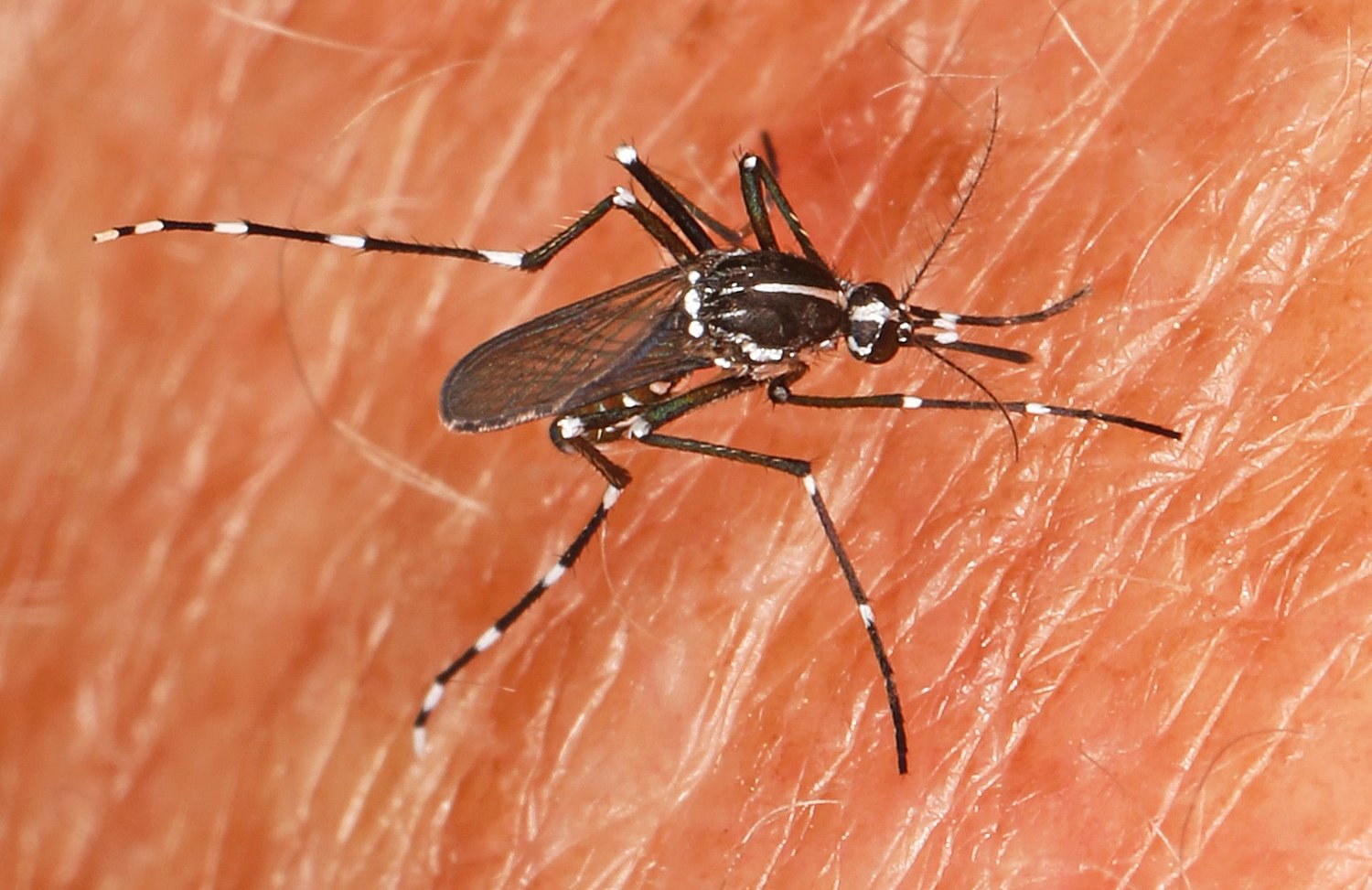This color photograph, taken with a macro lens, captures an extreme close-up of a black mosquito adorned with white accents as it bites into human skin. The highly magnified image reveals the intricate details of the mosquito's body: it has three long legs on each side, each adorned with white bands at the joints. A distinctive white stripe runs down its head and thorax, complementing the white dots that periodically appear across its back. The mosquito's head features two long, thin antennae that are feathery and spiky, along with a proboscis piercing the skin. The insect's slightly translucent wings are visible, extending back from its body.

The human skin, which occupies the entire background, appears peachy-pink with a rough texture, resembling a tan or pinkish-tan Caucasian skin. The skin's surface is detailed with numerous crease lines and sparse white hairs. The lighting and focus are so precise that every minute feature is visible, making the mosquito's markings and the skin's textures remarkably clear. The overall dominant colors in the image are the flesh tones of the skin and the contrasting black and white of the mosquito.